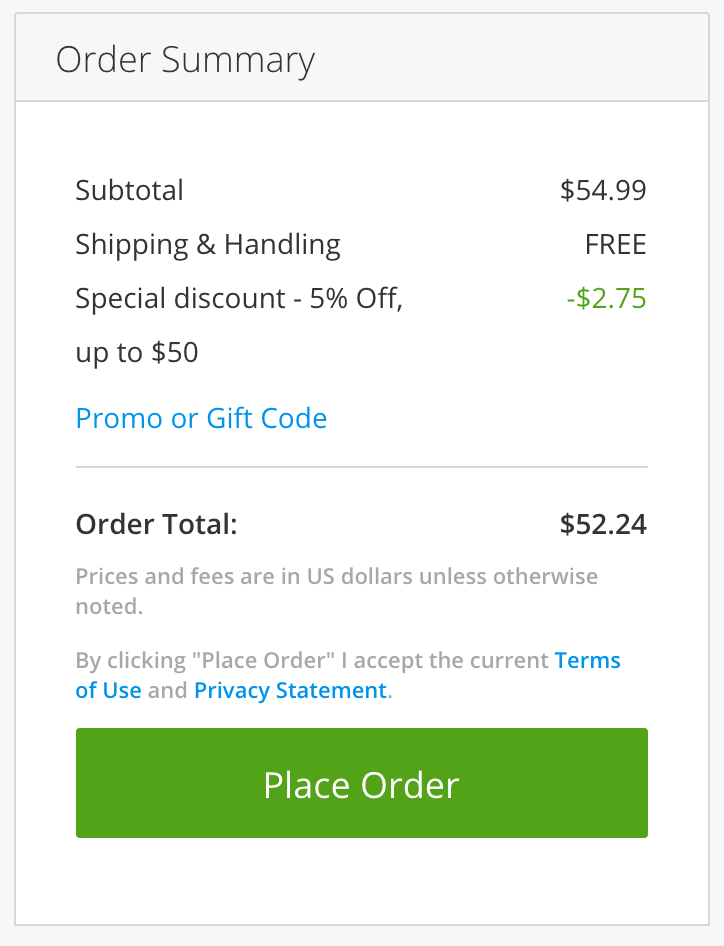A detailed caption for the described image:
---
The image depicts a mobile-optimized web page displaying an order summary, formatted to fit the narrow frame of a smartphone screen. The summary includes a subtotal of $54.99, followed by line items for shipping and handling, a 5% discount applicable to amounts up to $50, and a field for entering a promotional code or gift card. Below these details, the order total is calculated at $52.24, with a note specifying that all prices and fees are in US dollars unless otherwise stated. Underneath this, a disclaimer appears, stating that by clicking "Place Order," the user agrees to the terms of use and privacy statement—which are both hyperlinked for further review. The highlighted call-to-action is a green button labeled "Place Order" in white text, inviting users to finalize their purchase. The image does not specify the items being ordered or the website from which the order is made; it is solely focused on the final steps of the order confirmation process.